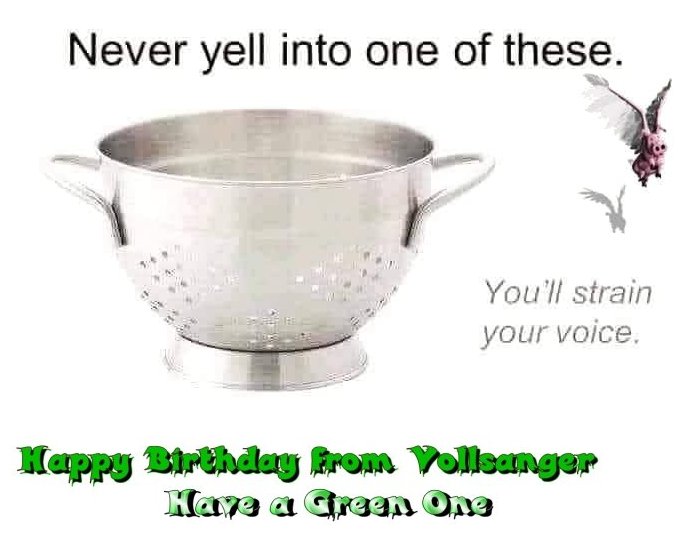The image features a centrally positioned metallic colander, often used for straining pasta or other foods cooked in water. This silver strainer has two wide handles near the top for easy tilting and drainage. The background is white, making the colander stand out prominently. On the right-hand side of the image, there's a whimsical drawing of a small pink flying pig with feathery white wings. The pig drawing is simplistic and lacks intricate detail. Above the colander, in black text, it humorously states, "Never yell into one of these." To the right of the colander, aligned with the pig, grey text continues the joke with, "You'll strain your voice." At the very bottom of the image, green text reads, "Happy birthday from Ballsanger," followed by the quirky wish, "Have a green one." These elements collectively suggest the image is a lighthearted, pun-filled birthday greeting.